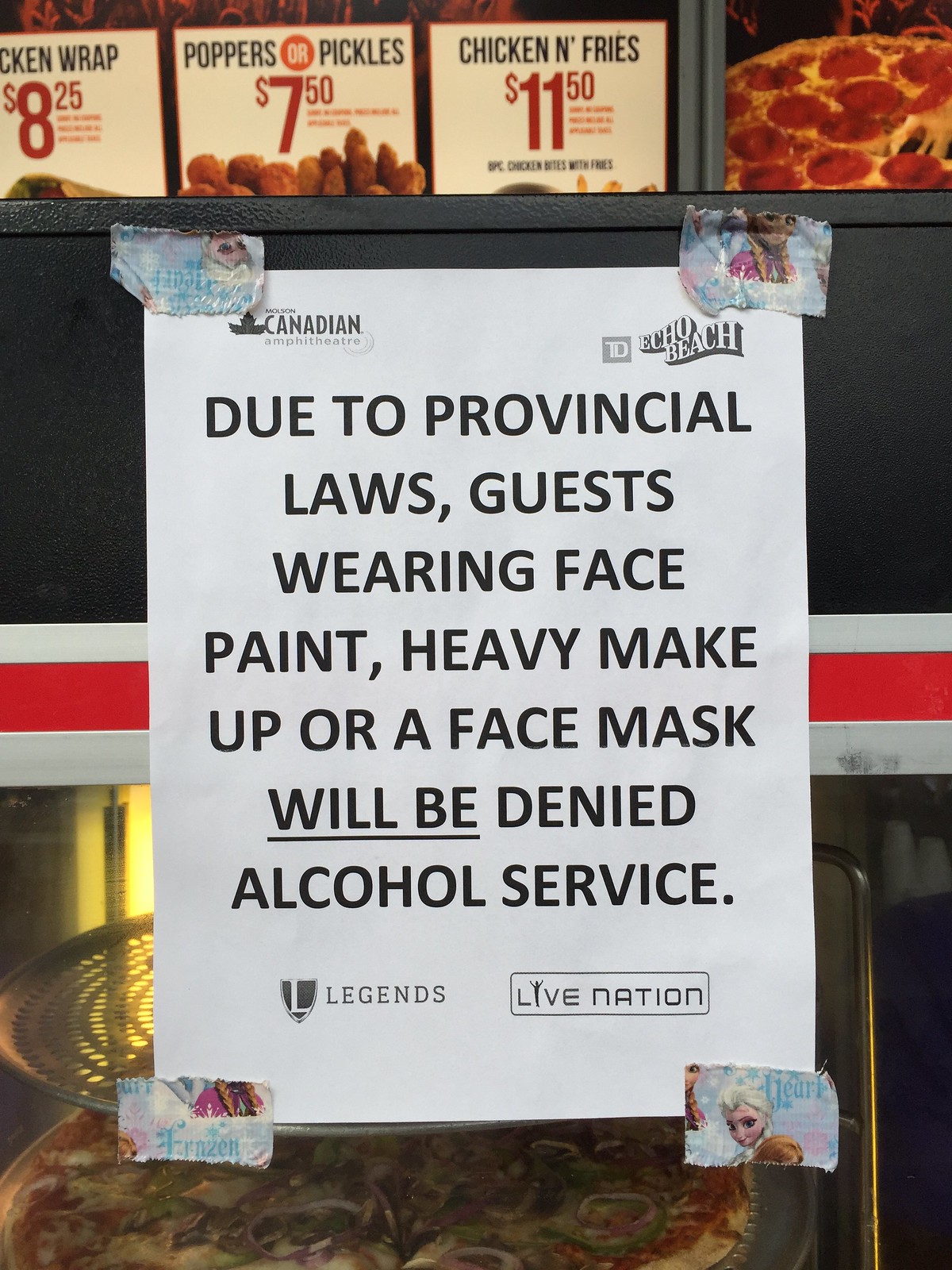The image captures a detailed scene inside a pizza shop where a white printer paper sign is prominently displayed on a glass wall, partially covering the display of a pizza. The sign is attached with tape featuring characters from the popular animated movie "Frozen" at its four corners. The sign informs patrons that due to provincial laws, guests wearing face paint, heavy makeup, or face masks will be denied alcohol service. Above the sign, a menu board hangs from the ceiling, advertising items such as chicken and fries for $11.50, poppers and pickles for $7.50, and a chicken wrap for $8.25. This detailed menu further indicates the establishment as a casual dining restaurant. Additionally, the context suggests this notice might be tied to an event managed by Legends and Live Nation at Echo Beach.